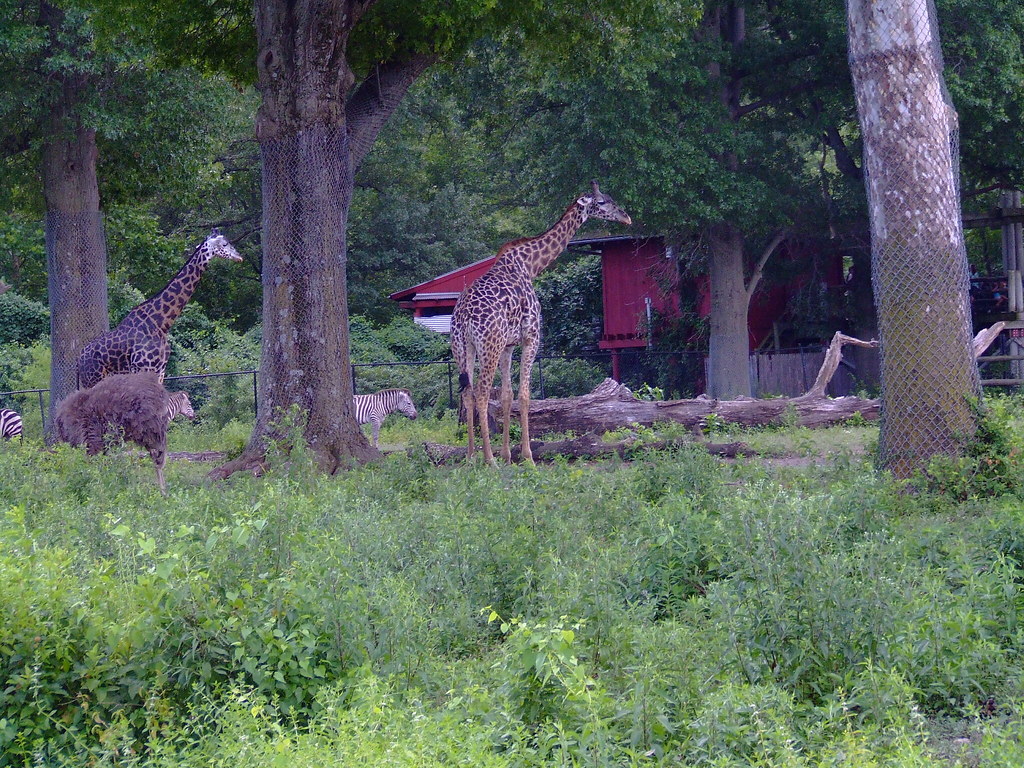The image depicts a shaded nature preserve within a zoo, characterized by lush greenery and various animal inhabitants. The foreground is abundant with knee-to-waist high green shrubs and wild grass. Several large trees tower in the background, along with a red barn-like structure, possibly a feeding storage area, flanked by robust fencing. A downed tree trunk lies mid-frame, enhancing the natural environment.

Central to the image are two giraffes, both looking towards the right. One giraffe is notably taller than the other, suggesting the presence of a juvenile. Nearby, two zebras are visible, with another zebra's hindquarters just making it into the frame on the far left side. Additionally, there appears to be a third zebra near the giraffes, partially obscured by the foliage. The area is enclosed by a black chain-link fence, with nets strung above adding to the authenticity of the habitat. The overall scene is richly shaded with lush green trees and bushes creating a vibrant, naturalistic backdrop.